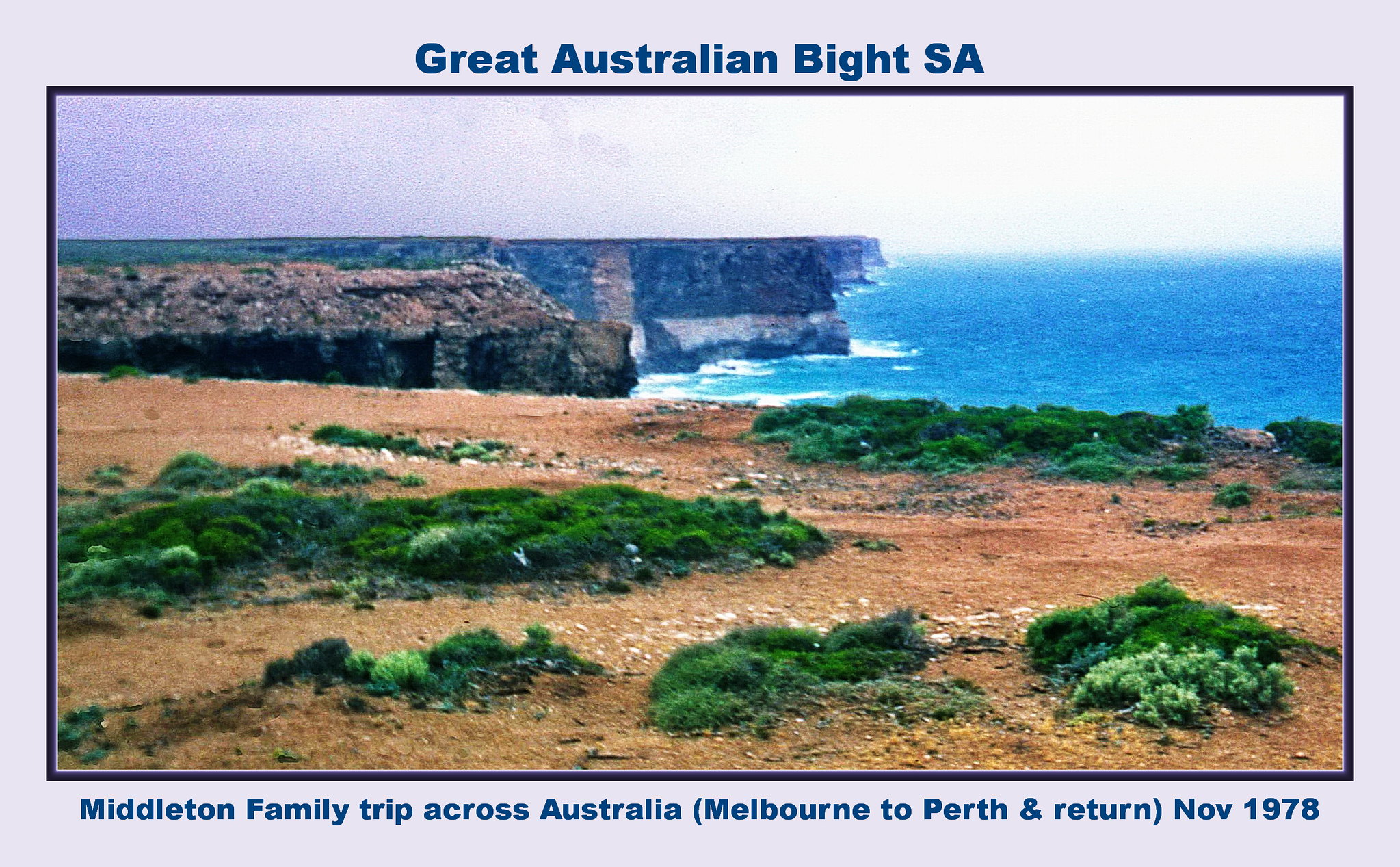This is a wide rectangular image that is digitally framed and captioned. The frame is wider at the top and bottom than it is on the left and right sides. It is a very light purple color with a dark purple inner border. The top of the frame features bold blue text that reads "Great Australian Bight Essay," while the bottom reads "Middleton Family Trip Across Australia (Melbourne to Perth and return), November 1978" in the same blue font. The photograph captures a striking scene of a rugged landscape. The bottom half reveals a light brown, sandy area interspersed with patches of thick, green grass and scattered rocks. The image highlights a central cliff that forms part of a series of larger cliffs. To the right, the vibrant blue ocean extends towards the horizon, with white waves crashing against the rocky coastline. The sky above is predominantly white, with overcast clouds suggesting an impending storm, particularly darker on the top left. The visual depth of cliffs to the left frames the expansive view, while the detailed textures of dirt and vegetation add contrast and richness to the scene.